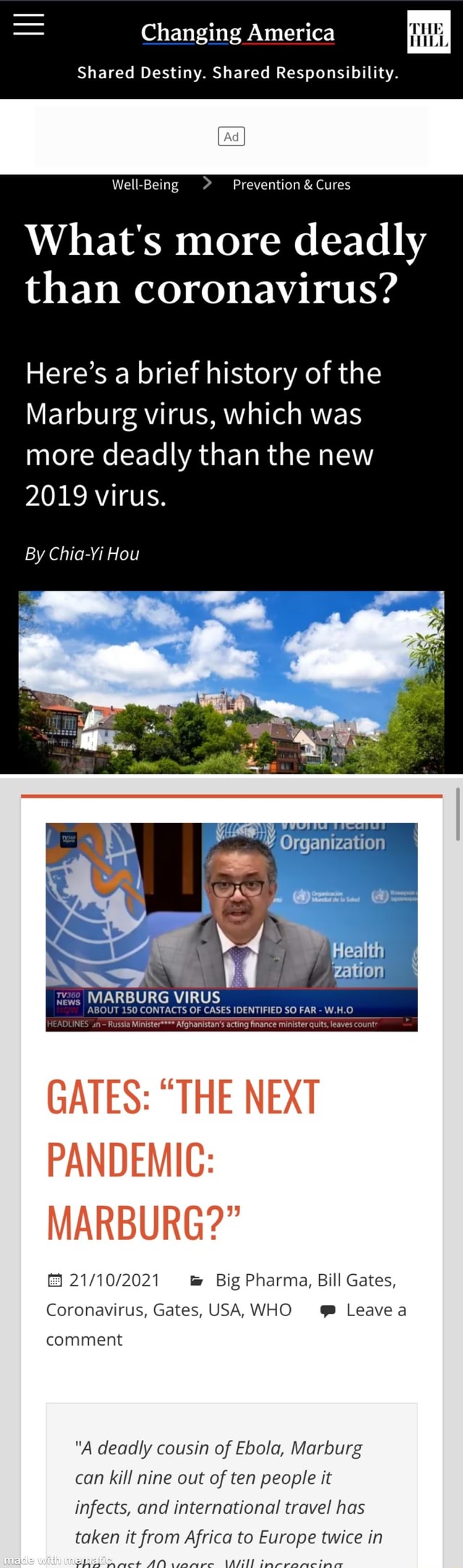Screenshot from "Changing America" on The Hill website showing a news headline and images related to the Marburg virus. The Hill logo is located in the bottom left of the screenshot, consisting of a white square with the words "The Hill" in black, spanning two lines. The news headline reads, "What's more deadly than coronavirus?" with a subheadline stating, "Here's a brief history of the Marburg virus which was more deadly than the new 2019 virus."

The screenshot also includes a background image of a picturesque hilltop town beneath a clear blue sky with scattered clouds. Below this, there's an image of the head of the World Health Organization. Superimposed on the images is a banner that reads, "Marburg virus: about 150 contacts of cases identified so far." At the bottom of the screenshot is text that references Bill Gates and mentions the "next pandemic" with "Marburg."